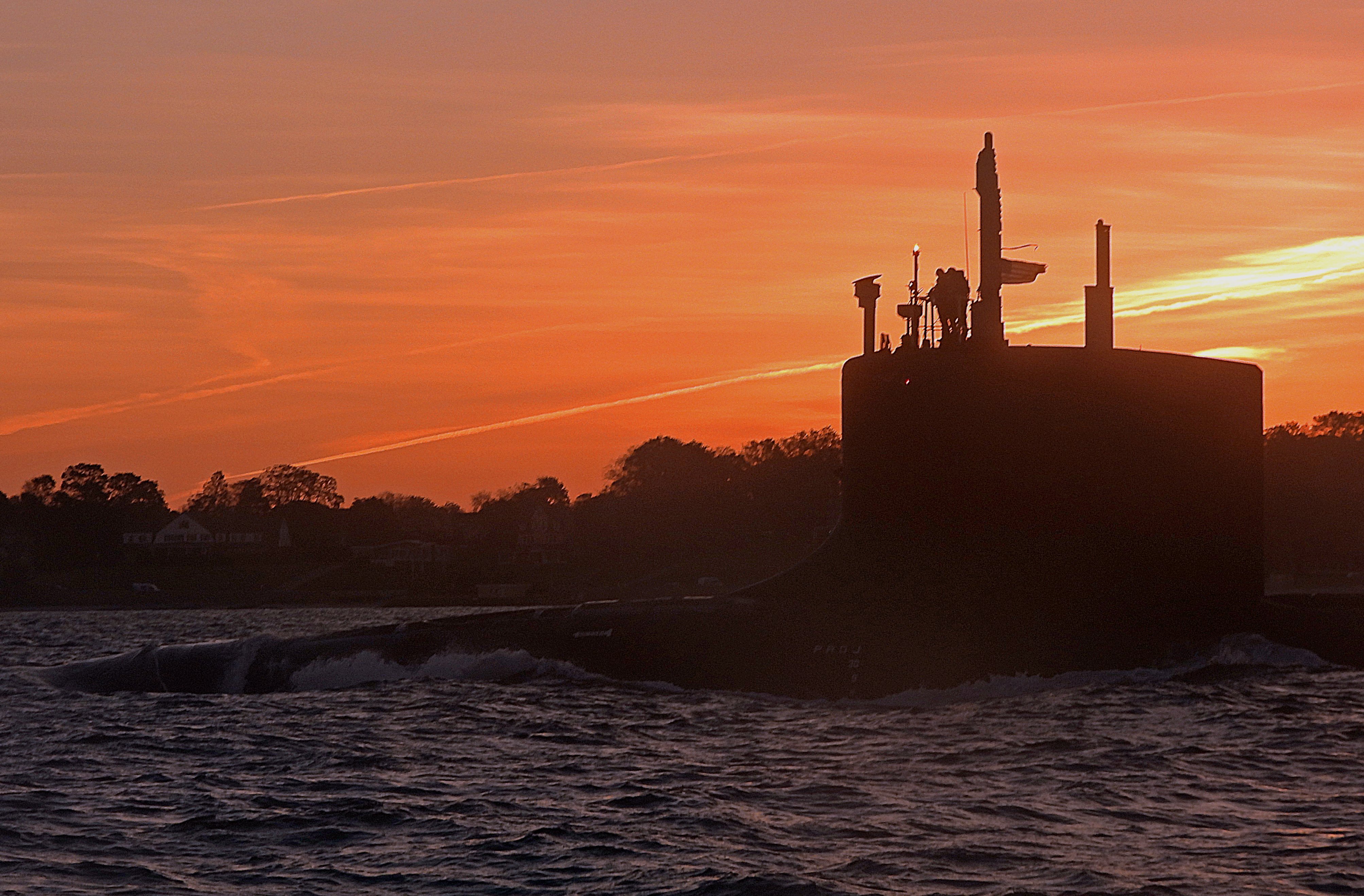The photograph captures a stunning outdoor sunset scene, with the sky ablaze in various shades of pink, orange, and deep red, accentuated by streaks of potential clouds. The foreground features a large body of slightly choppy water, with gentle waves creating a sense of movement. On the right-hand side, there's a dark, almost shadowy silhouette of a large industrial structure, potentially a submarine or an oil tankard, making its way through the water. This structure is difficult to detail due to the intense backlighting from the sunset, which creates a stark contrast. In the background, partially obscured by the silhouette and shadow, a treeline stretches across the image. Toward the center half of the photo, additional trees are faintly visible. There's also what appears to be a dock that extends from the water towards the industrial structure, traversing from the left to the right side. The interplay of light and shadow captures an atmosphere of serene yet powerful motion, underscored by the beauty of the vivid sunset.